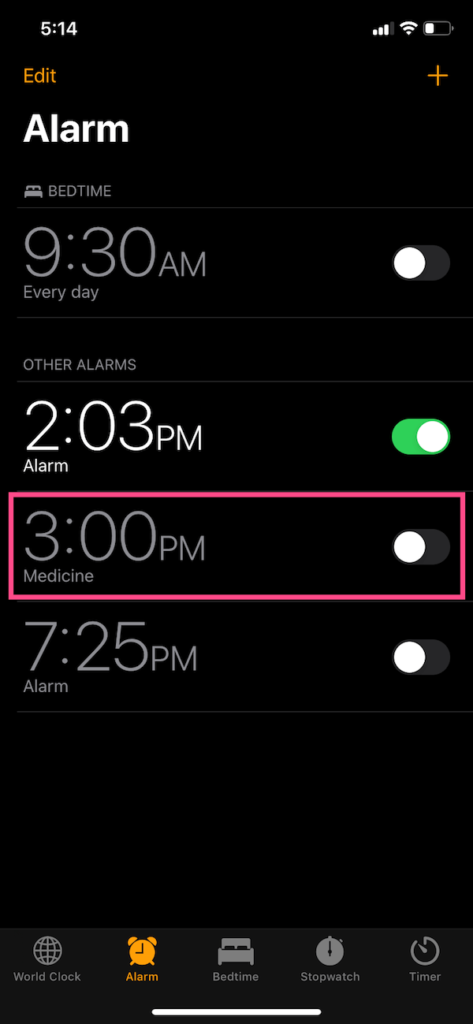This image depicts a screenshot of a smartphone's clock application, which is set to a dark theme for increased visibility and reduced eye strain. At the top of the screen, the time is displayed as 5:14, with full cellular signal bars, a strong Wi-Fi signal, and a quarter battery life remaining. The editing mode is activated, indicated by the yellow "Edit" button at the top.

On the right side of the screen, a plus sign allows the user to add new alarms. Below this, there is a list of set alarms: a recurring daily alarm at 9:30 a.m. that is currently turned on, as well as several other alarms, such as one for 2:00 or 3:00 p.m. which is active (highlighted in green), and additional alarms set for 3:00 p.m. and 7:25 p.m. that are not enabled.

At the bottom of the screen, there are navigation options including "World Clock," "Alarm," "Bedtime," and other functions like "Stopwatch" and "Timer." Currently, the "Alarm" section is selected, as indicated by the yellow highlight.

Overall, this image provides a detailed overview of the user’s alarm configurations and their phone’s status indicators.